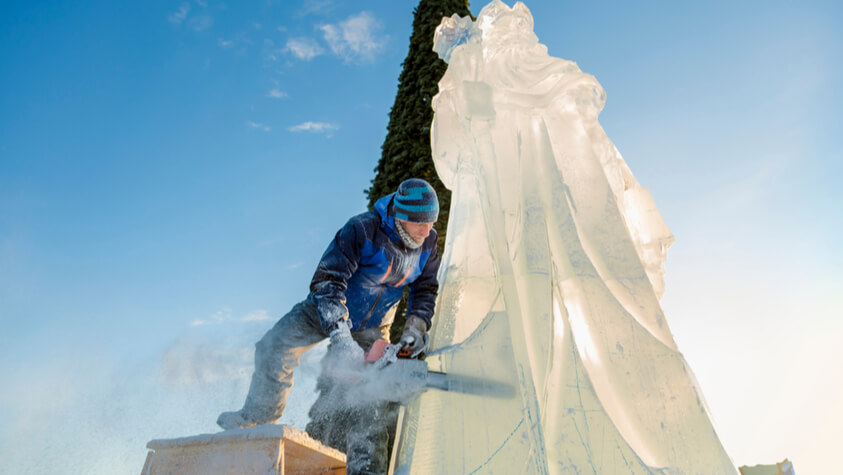In this outdoor winter scene, a man in winter clothing is meticulously working on an immense ice sculpture with a chainsaw. The sculpture, towering over the man who stands on a ledge to reach higher areas, depicts a robed figure with a flowing beard and a scepter. The artist, dressed in blue and black attire, including a jacket, snow pants, gloves, boots, and a blue and black knit beanie, stands amidst a sunny day with a mostly clear blue sky. His face is partially exposed, possibly covered by a turtleneck or face mask pulled down. An evergreen tree, perfectly triangular and towering, is visible behind the sculpture, set against the serene blue sky. The ice block, still largely uncarved, shows intricate initial detailing of the robed figure, promising an elaborate artwork once finished.